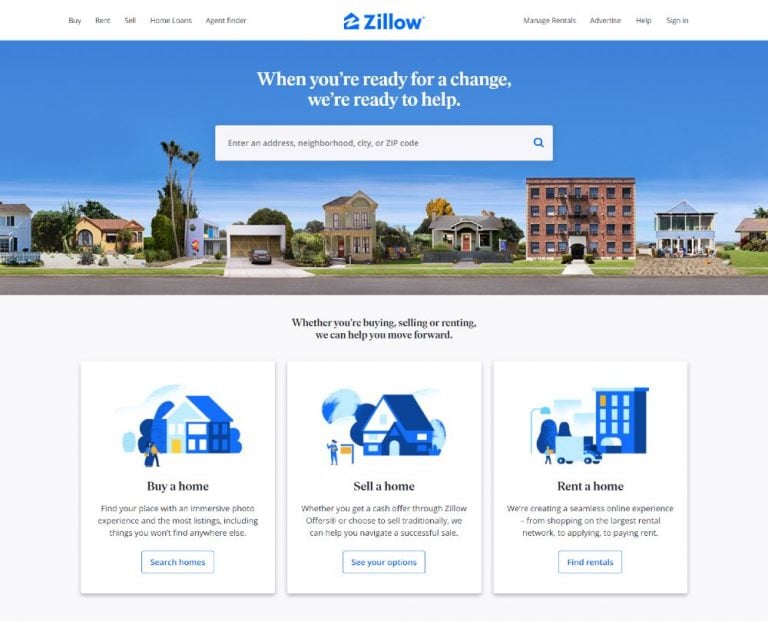The image, sourced from Zillow, is meticulously structured and visually appealing. 

At the top of the image, there's a white border bearing the prominent, bold blue text "Zillow," accompanied by the Zillow logo on the left. Adjacent to the logo, moving from left to right, are navigational options: "Agent Finder," "Home Loans," "Sell," "Rent," and "Buy." On the right side of the "Zillow" text, the options continue with: "Manage Rentals," "Advertise," "Help," and "Sign In."

Directly below this top section, the image displays a picturesque neighborhood scene occupying the upper half of the page. The background features an idyllic bright blue sky. In the foreground, there is a sequence of houses: a white house, then a brown house, followed by another white house with a car in its driveway, another brown house, a green house, a substantial four-story concrete building, and finally, a blue house. These homes are set against a road in front, a grassy expanse between them, and trees in the background. Overlaying the sky, bold white text reads, "When you're ready for a change," with a follow-up line underneath stating, "We're ready to help."

Beneath this visual, a white search bar is positioned, featuring a search icon on the right side. The placeholder text within the search bar reads in black font, "Enter an address, neighborhood, city, or zip code."

The bottom half of the image is framed by a light grayish border. Centrally placed in black lettering, the text reads, "Whether you're buying, selling, or renting," with "We can help you move forward" displayed below.

At the very bottom are three white squares, each containing a blue illustration of different types of homes: the first is a two-story home, the second is a single-story home, and the third is a large building with a blue truck parked outside. Below each drawing, bolded black text identifies the actions: the first square says "Buy a Home," the second says "Sell a Home," and the third says "Rent a Home." Under each heading, three lines of detailed information are provided. At the bottom of these squares are white tabs with blue lettering indicating specific actions: the first tab reads "Search Homes," the second "See Your Options," and the third "Find Rentals."